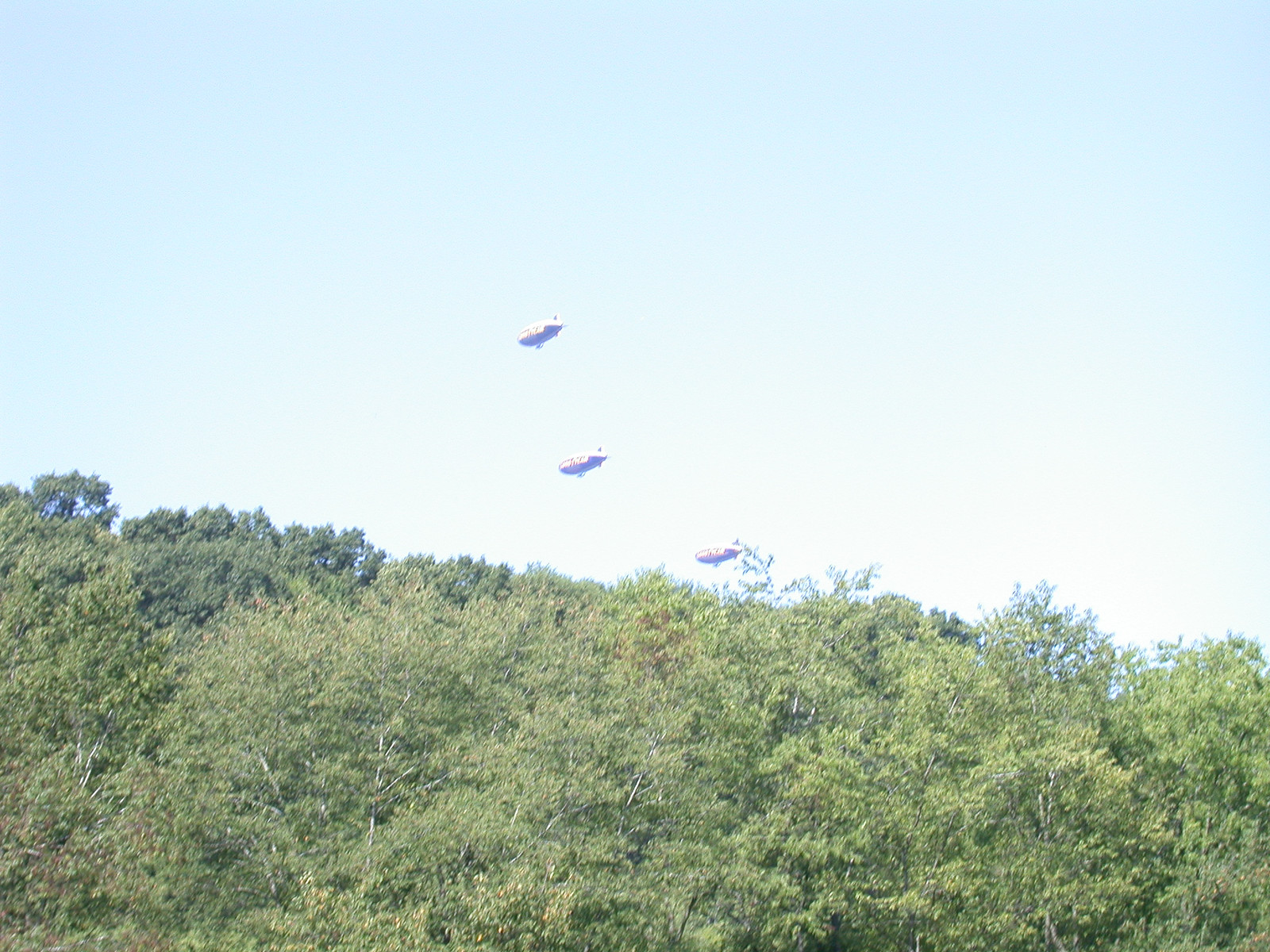In this vibrant outdoor photograph, three blimps gracefully hover in a clear, bright blue sky devoid of clouds. Below them, a dense forest of lush green trees extends across the bottom of the image, with no visible gaps between the foliage. The blimps are staggered in height, with the highest one positioned above the others. Each blimp features a white top and a darker, grayish bottom, appearing almost circular with prominent fins on the back and small cabins below for navigation. One crucial detail is the yellow "Goodyear" lettering displayed on each blimp's side. This picturesque scene captures the blimps floating harmoniously over the serene, green expanse of the forest.